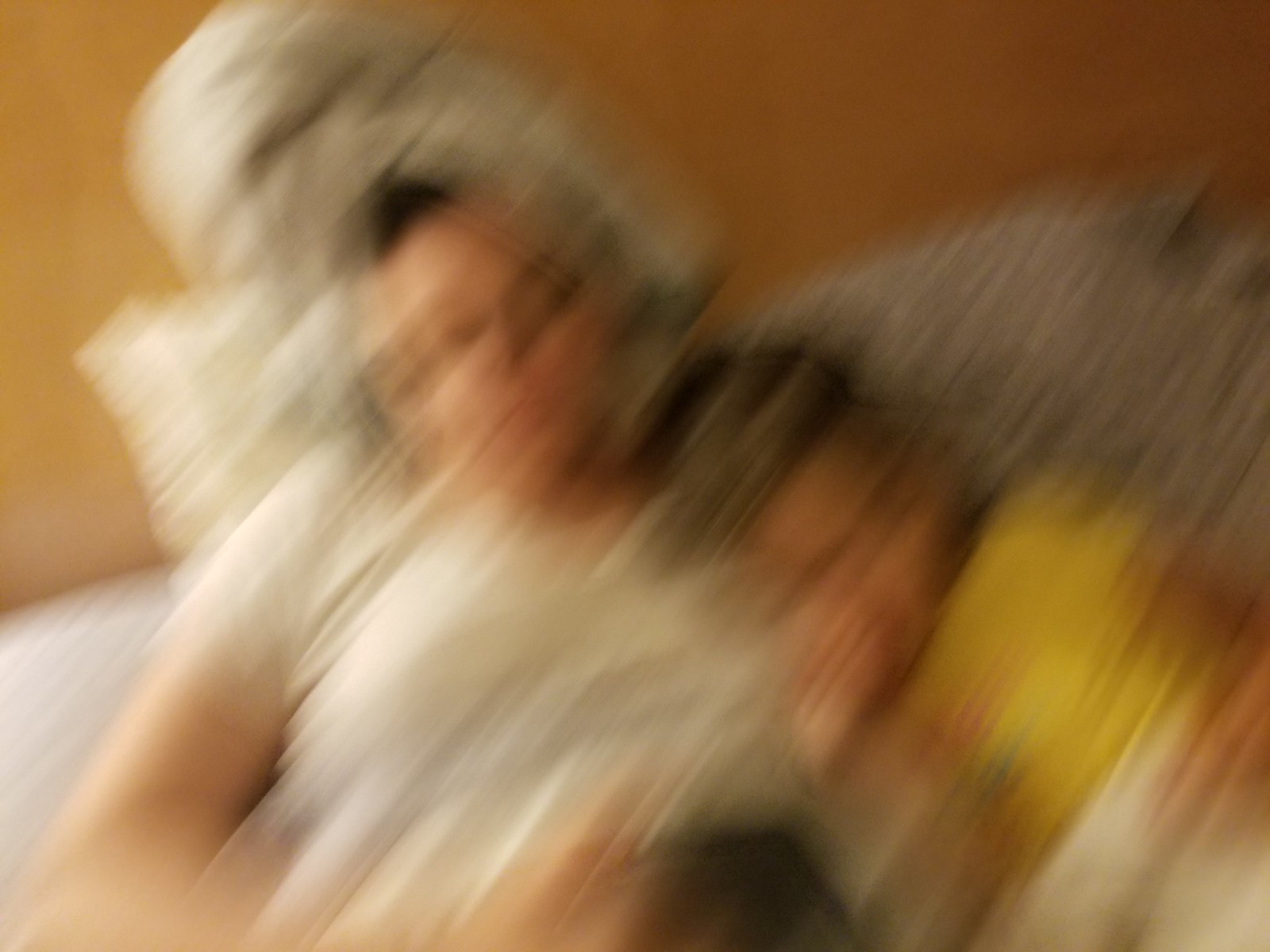This color photograph, though extremely blurry and lacking in fine detail, seems to depict a tender moment between a woman and a child. Central to the image, the woman is lying down, wearing a light white short-sleeved t-shirt and a wrap on her hair that looks to be white or possibly gray. There is a pillow positioned behind her right shoulder, and the backdrop features an orange wall to her left and our right. Nestled into her left shoulder is a small child, who appears to be resting their head there, with their hand close to their mouth. The child wears a short-sleeved yellow t-shirt adorned with a green and yellow logo or writing and light-colored trousers or a skirt. The pillow behind them has a darker, greyish hue, providing contrast to the scene. Additionally, a shadow can be seen near the right side of the woman's arm, situated between her and the child, adding depth to their intimate setting on what seems to be a couch or a bed.